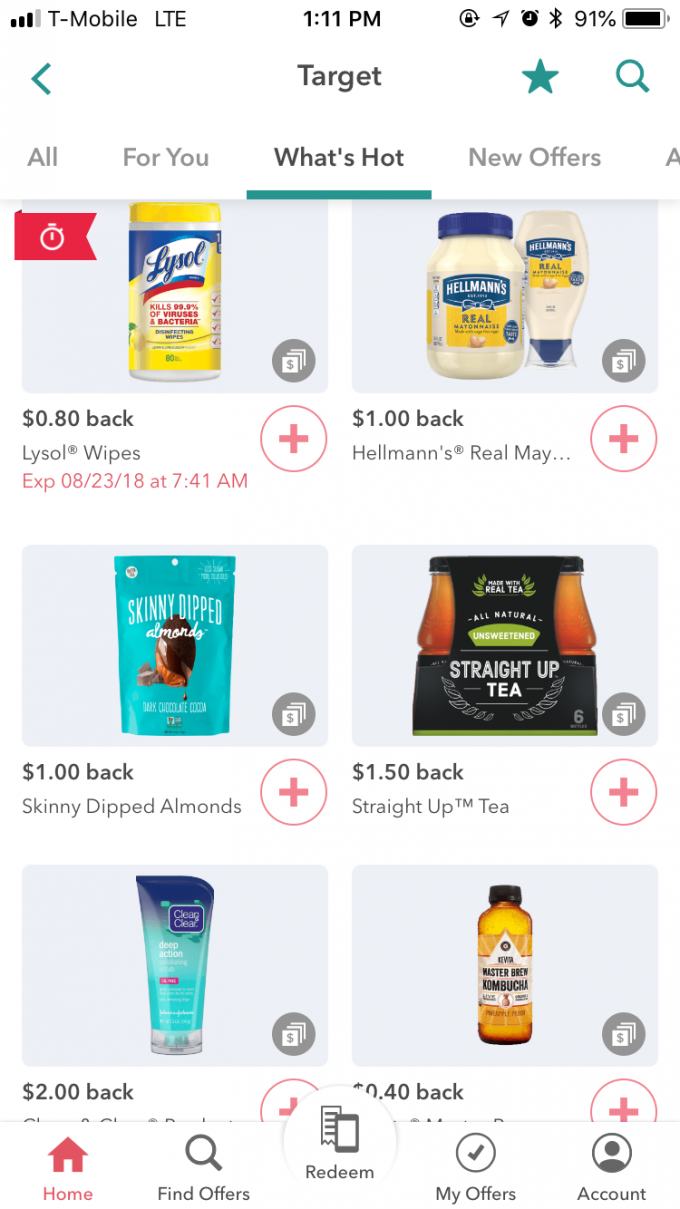The image features a user interface with various elements and product offers. 

At the top center, the word "target" is displayed in a bold dark gray font. Just to the left of the word "target," there's a teal arrowhead pointing left. To the right of "target," a bolded teal star is visible, followed by a magnifying glass icon with its top slanted to the upper left.

Below this interface, several options are presented in gray. The first option reads "all," followed by "for you," and "what's hot," which is currently selected, indicated by its darker font and a thick green underline. The next option is "new offers," also in gray, and there are additional options visible, though they are cut off after an "A."

The image then showcases several items. The first item is a pack of Lysol wipes, with the package colored in yellow against a light gray background. In the upper left corner of this section, a red tag featuring an alarm symbol indicates that the deal is expiring soon. At the bottom, there's text stating "$0.80 back" in bold, and below that, in gray text, it says "Lysol wipes." Further down, in red text, it states "exp 08/23/18 at 7:41 a.m." Next to this, there is a circle with a red border containing a bold red plus sign in the middle.

To the right, there is a section featuring Hellmann's mayonnaise. This includes a large jar and a squeezable jar behind it. Below these jars, it says "$1.00 back" in bold black letters. Further down, in gray lettering, it displays "Hellmann’s®," and beneath this, it says "Real May..."